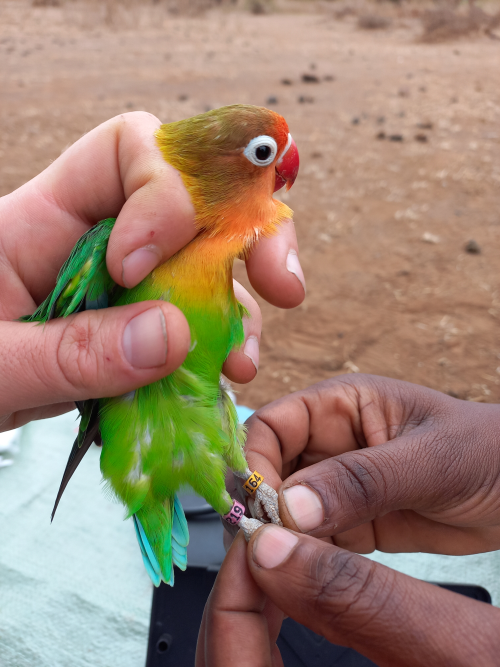This photograph captures a vibrant baby parrot being handled by three hands amidst a natural setting. The bird, likely a young parakeet, showcases an array of bright colors: a burnt-orange head, a distinct red beak, a white ring encircling its black pupil, orange feathers near its head, a green midsection, and an underside with both turquoise and green feathers. The bird's wings are gently secured by a pale hand emerging from the left side, holding it by the back and wings, while two brown hands from the lower right grasp each of its feet. The bird's ankles are adorned with two identification labels: one purple and one yellow, both inscribed with black numbers, suggesting it may be tracked or studied. They appear to be over a tarp-covered area, hinting at a research or conservation setting in the wild.